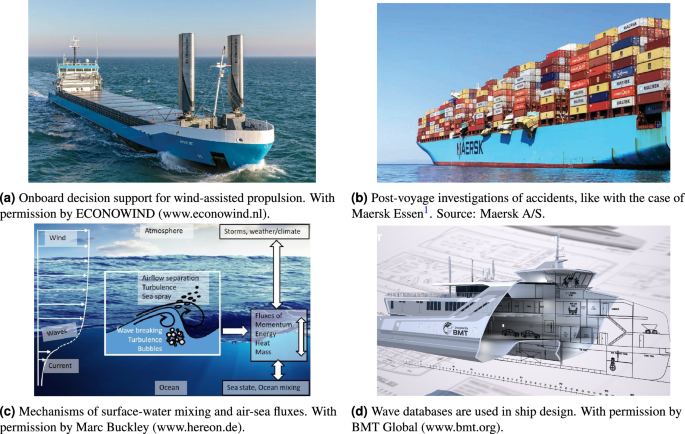This is a detailed screenshot of a slide featuring four images, each with distinct labels and captions. In the top left corner (A), there's an image of a long blue boat on the sea, accompanied by the caption "Onboard Decision Support for Wind-Assisted Propulsion" with permission from Econowind, and the link www.econowind.nl. The top right corner (B) features a large blue cargo ship labeled HRSC, loaded with numerous cargo containers in various colors; below this image is the caption "Post-Voyage Investigations of Accidents, like with the case of Maersk-Essen," sourced from Maersk A/S. In the bottom left corner (C), there's a graphic showing water and wave dynamics, accompanied by the caption "Mechanisms of Surface Water Mixing and Air-Sea Fluxes," with permission from Mark Buckley, and the link www.herion.de. The bottom right corner (D) displays a mixed 2D and 3D diagram of a boat, with the caption "Wave Databases are Used in Ship Design," with permission from BMT Global, and the link www.bmt.org.